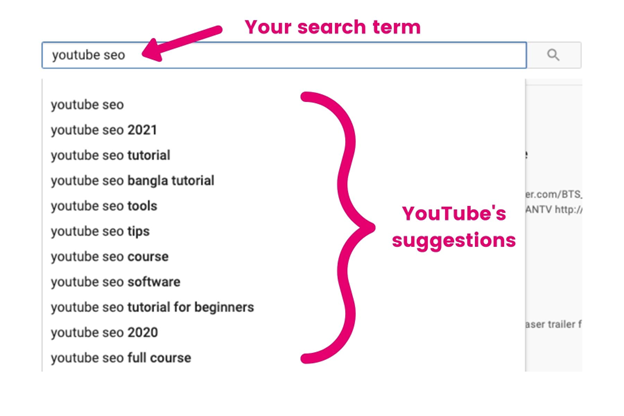This image illustrates a search query for "YouTube SEO" on the YouTube platform. The phrase "YouTube SEO" is highlighted with an arrow pointing towards the YouTube search bar. Below the search bar, a dropdown menu is shown, displaying various YouTube search suggestions. These suggestions include "YouTube SEO," "YouTube SEO 2021," "YouTube SEO tutorial," "YouTube SEO Bangla tutorial," "YouTube SEO tools," "YouTube SEO tips," "YouTube SEO course," "YouTube SEO software," "YouTube SEO tutorial for beginners," "YouTube SEO 2020," and "YouTube SEO full course." Each of these suggestions is framed with a tag that indicates they are YouTube's autocompleted suggestions. The image predominantly uses a red and black color scheme set against a white background, contributing to a clean and crisp visual representation.